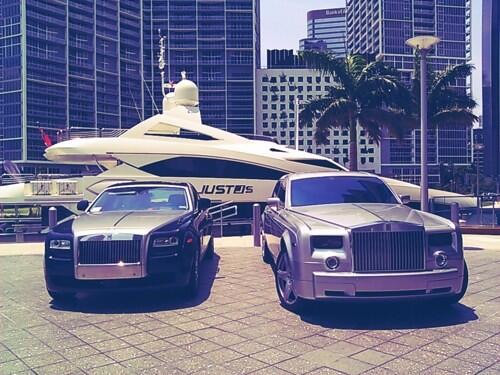In a vibrant, urban waterfront setting reminiscent of Miami, two luxurious Bentleys are parked on a stylishly sectioned marble-like pavement. The car on the right, a sleek silver model with a large grille, exudes sophistication, while the car on the left flaunts a striking combination of black and silver, with its silver bonnet and grille bordered by black details around the headlights. Both vehicles sit elegantly in front of a modern, two-level white yacht marked with the black letters "J-U-S-T-O-S." This spacious yacht features a sporty design and a distinctive red flag at the rear. In the background, towering skyscrapers with blue-tinted windows rise into a gray, cloudy sky, interspersed with a smaller white building. Nestled behind the yacht, a picturesque scene unfolds with palm trees and a streetlight, completing this image of opulent serenity.